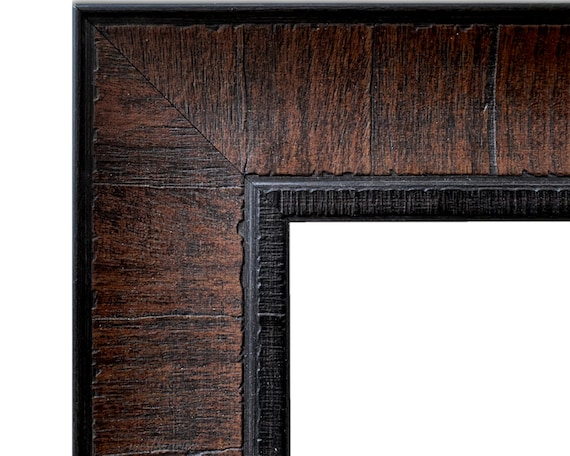The image depicts a close-up of the corner of a frame, forming an inverted L shape, oriented 90 degrees to the right. The frame appears to be constructed from dark brown wood, exhibiting various shades of brown with darker areas that seem intricately etched. The inner edge of the L-shaped frame is outlined in black, which has a textured appearance that might be wood or a wood-like plastic. The background of the image is white, providing a stark contrast that highlights the frame's detailed grain patterns and layered design features. This partial view focuses primarily on the upper and left sections of the frame, allowing a detailed inspection of its composition.